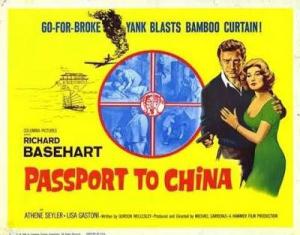The image is a vintage movie advertisement on a bright yellow background from what seems to be the 40s or 50s. Central to the poster are a man and a woman. The man, with brown hair, is dressed in a black sweater over a white shirt, holding a revolver in his right hand. His arm is wrapped protectively around the woman, who has short blonde hair and is wearing an elegant green dress, her left hand resting on the man's chest, looking slightly scared. At the top of the poster, in black font, it reads "Gopher Broke Yank Blast Bamboo Curtain," and below that is the name Richard Baseheart. Dominating the lower part of the advertisement is the movie title "Passport to China" in bright red font. A prominent circle resembling a gun sight, featuring red and blue elements, is central to the image, adding a sense of action and suspense. Off to the side, there's an airplane trailing thick black smoke, suggesting it may be crashing, possibly into a depicted building. The corners of the poster are adorned with black and white images, enhancing the dramatic feel of the advertisement.